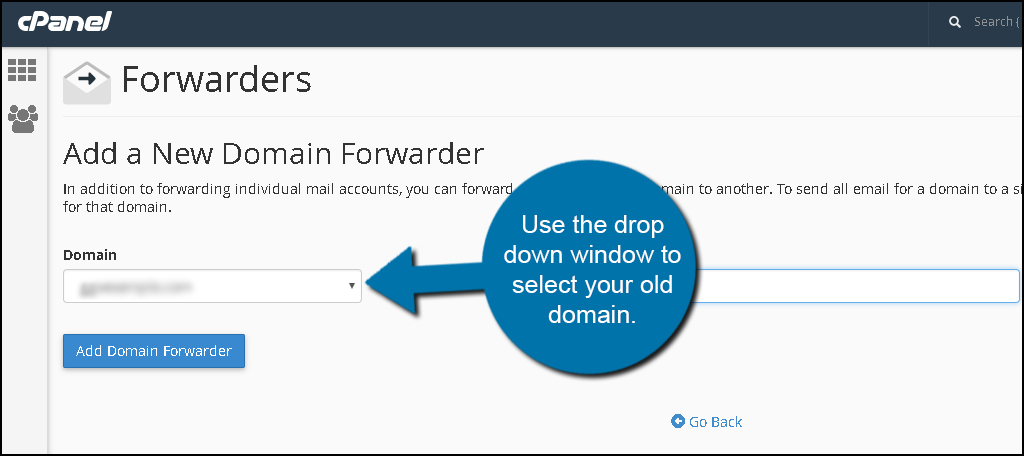This web page features a user interface dedicated to managing email forwarders. At the top of the page, there is a blue header with the word "Panel" displayed in white text on the left side. On the right side of the header, there is a "Search" label accompanied by a magnifying glass icon. 

In the central section of the page, the word "Forwarders" is prominently displayed. Adjacent to this word is a symbol of an envelope with a right-pointing arrow, indicating the email forwarding function. Below this, the phrase "Add a New Domain Forwarder" is visible. The text underneath attempts to explain that users can forward all email from one domain to another domain. However, part of this text is obscured, reading: "...in addition to forwarding individual mail accounts, you can forward...the rest of the words in the center are obscured...and after it says main to another to send all email for a demo domain to a SI for that domain."

In the center of the interface, there is a large, blue, round circle with an arrow pointing to the left. This circle contains the instruction: "Use the drop-down window to select your old domain," and it points towards a drop-down window labeled "Domain." The contents of the search bar next to this drop-down are blurred out. Below the drop-down, there is a blue box with the text "Add Domain Forwarder" written in white.

Additionally, under the large circle, there is a smaller circle with an arrow and the words "Go Back" written in blue. This icon offers a navigation option to return to the previous page.